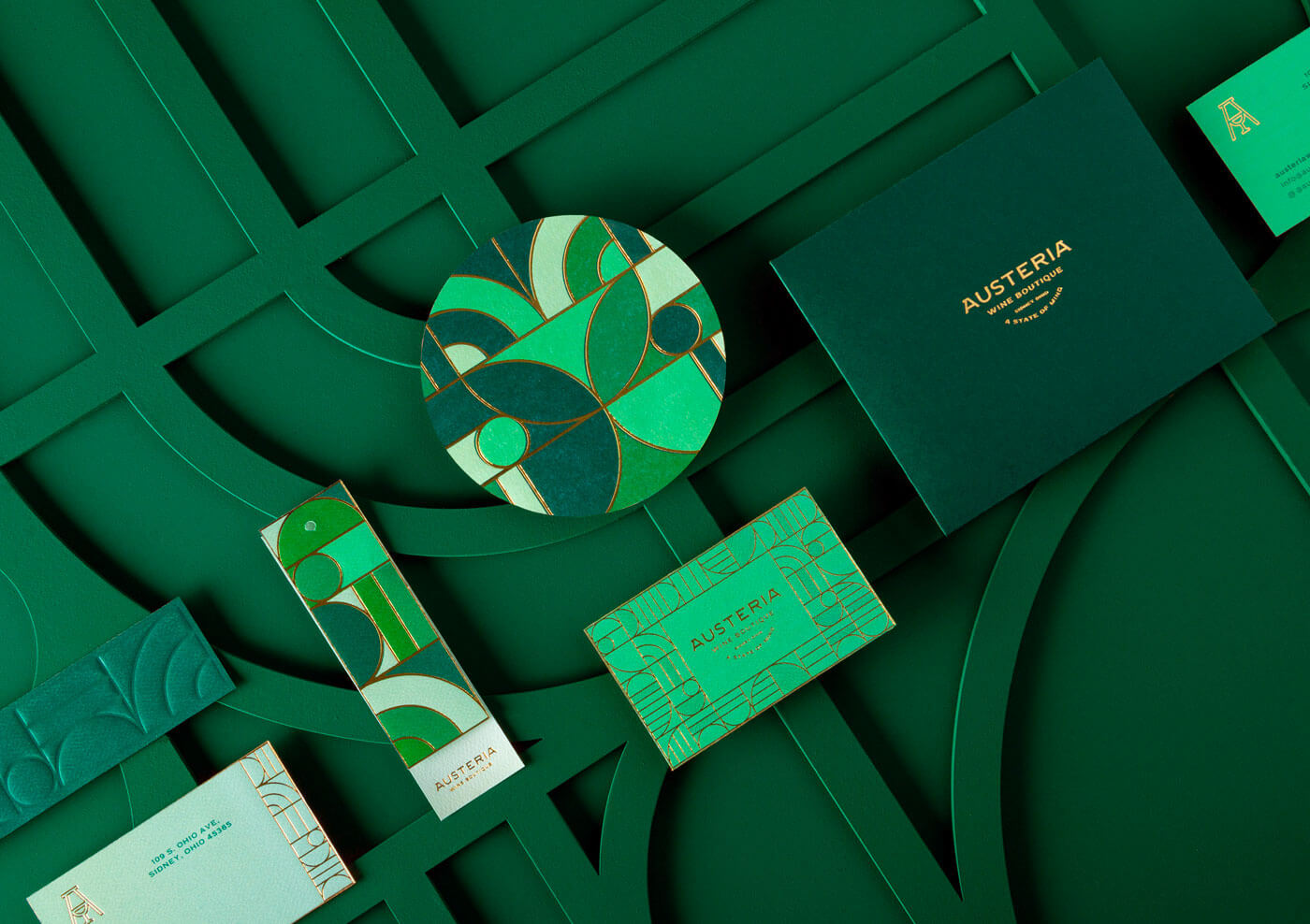The image features a visually stunning advertisement shot set against a forest green background with an embossed pattern of intersecting curved lines and geometric shapes. The backdrop, reminiscent of brocade, adds a touch of elegance. Various green-themed objects are meticulously arranged on top, contributing to a cohesive aesthetic. On the far right, a light green box showcases a white logo in the upper left corner. Adjacent to it, a dark green box with gold lettering prominently displays the word "Austeria" on its top line. In the center, a round disc adorned with a modern art geometric design in shades of forest green, mint green, and white captures attention. Beneath the disc, a mint green label also bears the name "Austeria." To the left, a longer, portrait-oriented rectangle continues the consistent color scheme and repeats the "Austeria" branding. In the bottom left corner, a very dark green quilted box and a white label with illegible writing complete the arrangement. Collectively, these items, possibly jewelry boxes and promotional materials, emphasize the recurring gold and green theme, potentially promoting "Austeria Wine Boutique."